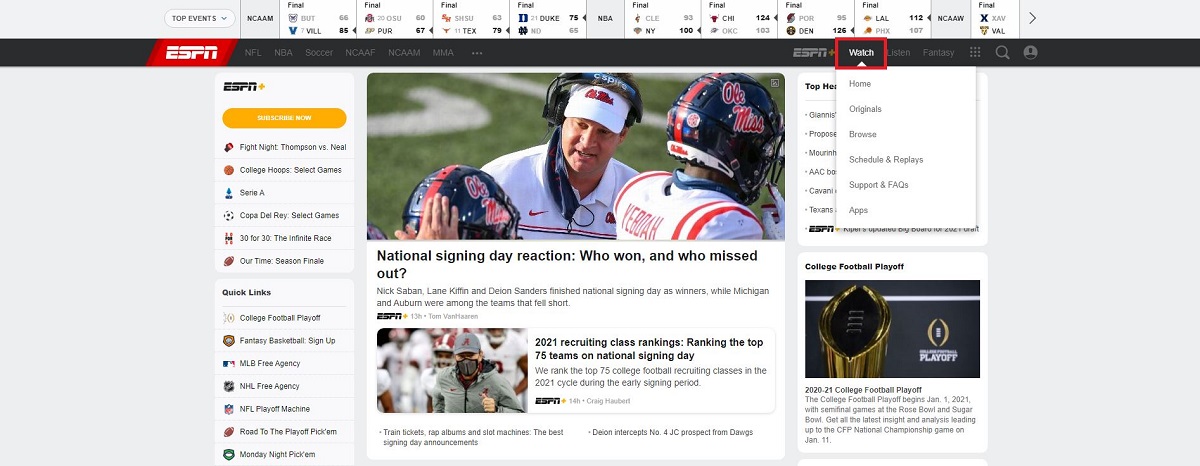### Detailed Caption:

The image is a screenshot of an ESPN web page, prominently displaying a listing of sports events and game outcomes at the top. The section includes final scores from both college teams and professional leagues. Notable game scores are as follows: Final score between Butler and Villanova with VILL85 and BUT66, Ohio State versus Purdue ending OSU60 to PUR67, Sam Houston State against Duke with SHSU63 and Duke75, and Notre Dame at ND65 in the NBA scores segment, notable scores include Cleveland at CLE93 against New York at NY100, Chicago at CHI124 versus Oklahoma City at OKC103, Portland at POR95 with Denver at DEN126, Los Angeles Lakers at LAL112 against Philadelphia at PH6107. In the NCAAW section, one game shows a final outcome but the scores for XAV and VAL are not visible.

On the left-hand side of the webpage, a vertical navigation bar is present. At the top, it displays the ESPN logo alongside an orange "Subscribe Now" button. Below this, there are clickable options such as Fight Night featuring Thompson vs. Neal, College Hoop with Select Games, Serie A, Copa del Rey with Select Games, the 30 for 30 documentary "The Infinite Race", and "Our Time" Season Finale. Quick Links provide access to various sporting activities and sign-ups, namely the College Football Playoff, Fantasy Basketball, MLB and NHL Free Agency, NFL Playoff Machine, Road to the Playoff Pick'Em, and Monday Night Pick'Em.

Additionally, an image is included on the webpage showing a coach dressed in white, engaged in a discussion with two football players donning white jerseys with red stripes and black helmets featuring a red stripe.